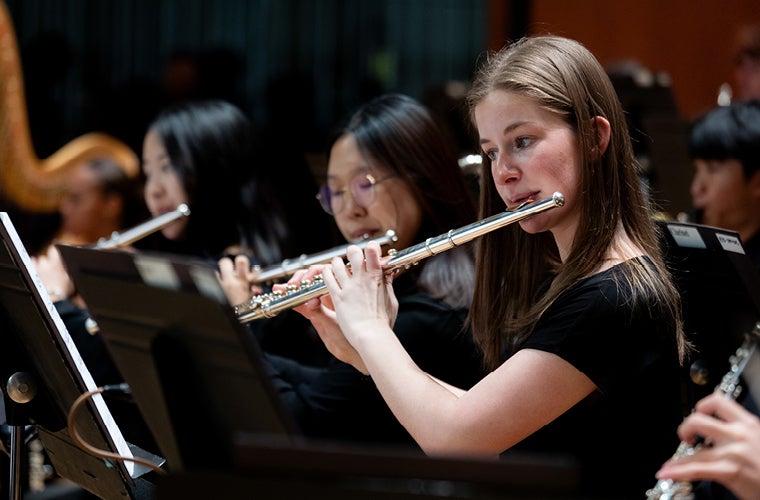This close-up, indoor photographic image captures the intense focus and collaboration of an orchestra playing what is likely classical music. Central to the composition are three female musicians engrossed in their performance, each playing a silver flute. 

On the far left, slightly out of focus, is an Asian woman with long black hair, her eyes intent on the music. To her right stands another Asian woman, distinguishable by her silver-framed glasses and long black hair, also playing a flute. Dominating the center of the photograph is a white woman in her late teens or early twenties, with long brown hair and a short-sleeved black dress or shirt, which reveals her arms as she looks downward, concentrating on her flute.

In the detailed periphery of the image, the fingers of another musician playing what appears to be a clarinet can be seen in the bottom right-hand corner. Behind the flutists, the background reveals further layers of the orchestra, including blurred figures and indistinct instruments. The setting features orange walls and green curtains, providing a warm and complementary backdrop.

Additional details include a harp emerging from the top left corner, its brown or goldish outline visible, and another Asian individual playing a woodwind instrument faintly seen in the top right corner. A music stand with a white book on it is positioned in front of the musicians, framed in black and silver and held up by a pole. This richly detailed image captures the harmonious yet intricate essence of an orchestral performance, with every element contributing to the overall ambiance.